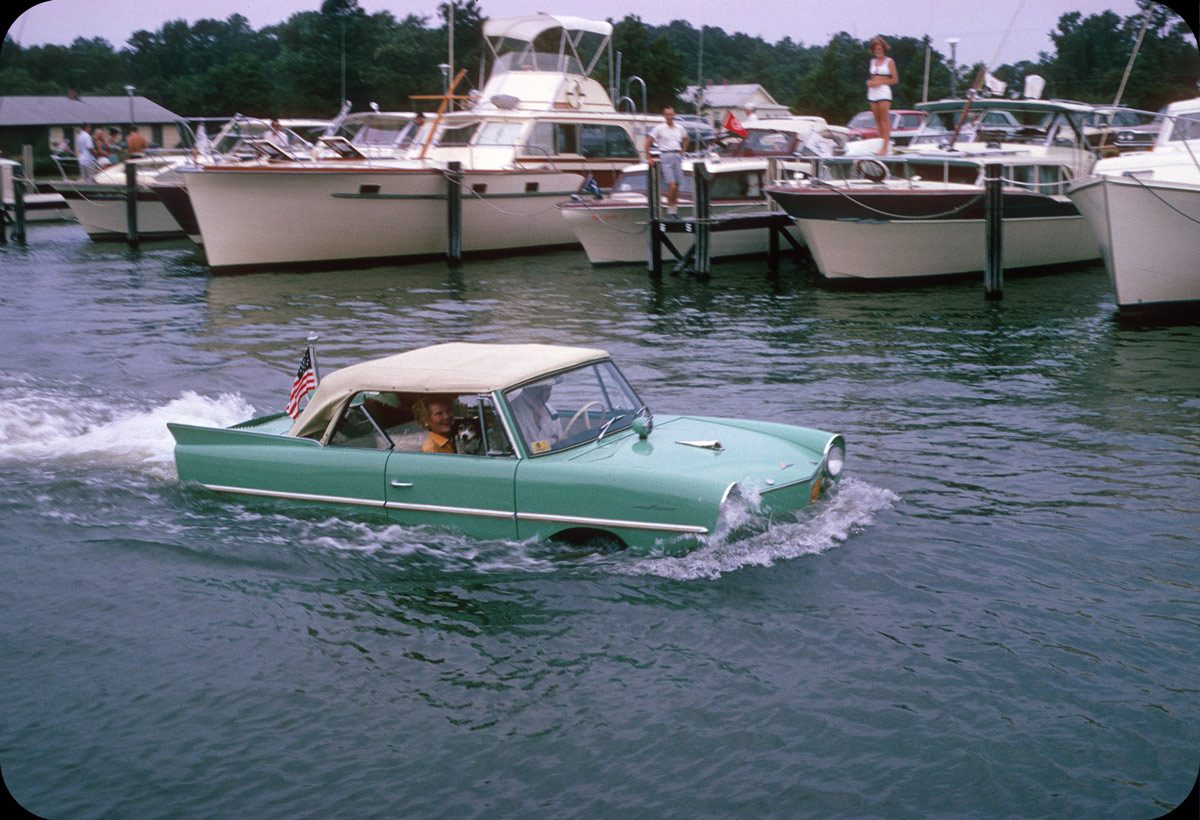The image depicts a unique scene of a classic mint green 1965 Amphicar Model 770, an amphibious vehicle, driving through a body of water that appears to be a lake or river. The car, which has a white convertible top and detailed chrome trim—including a chrome pinstripe, handles, and headlight bezels—is in motion, creating noticeable ripples and frothing water behind it. The license plate boasts a small American flag. Inside the car, a man is at the wheel, accompanied by his wife, who is holding a small black and white dog on her lap. The scene takes place on an overcast, hazy day. In the background, a row of docked sailing boats and yachts can be seen, with people aboard watching the extraordinary spectacle. Behind the boats, a tree line is visible under the light gray sky, adding depth to the image. The water reflects a deep blue-green hue, enhancing the picturesque setting.